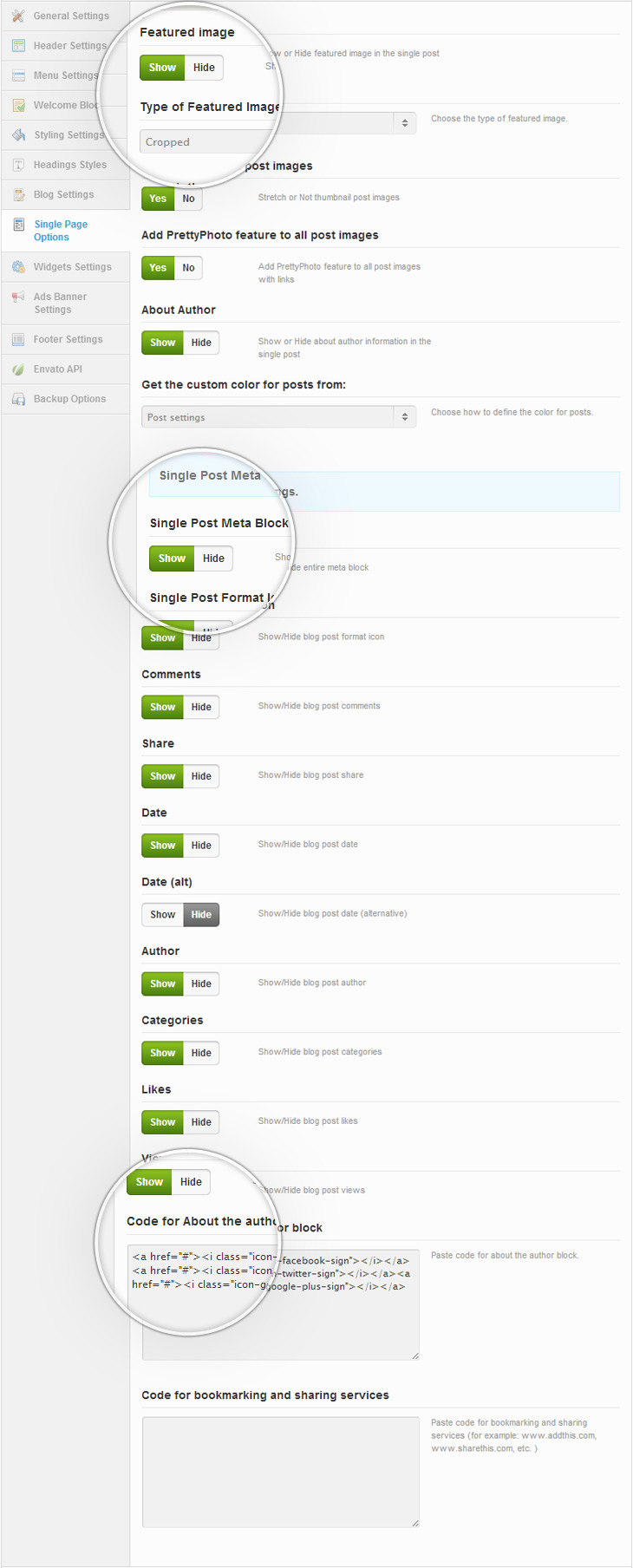This screenshot depicts the General Settings page of a computer interface, organized into two main sections. 

On the left-hand column, there are several icons accompanied by their respective labels displayed in vertical order. The text includes: 

- General Settings
- Header Settings
- Menu Settings
- Welcome Block (partially covered by an image)
- Style Settings
- Headings
- Styles
- Blog Settings
- Single Page Options
- Widget Settings
- Ad Spanner Settings
- Footer Settings
- Envato API
- Backup Options

On the right-hand side of the page, the section starts with "Featured Image" in bold, where the "Show" tab is highlighted, indicating its active status. Below this, the subsection "Type of Featured Image" is shown with the option "Cropped" selected in the corresponding menu. Over this area, there's an overlay of a magnifying glass icon.

Further down, there is an option stating "Stretch or Not Thumbnail Post Images," which is enabled. Another setting labeled "Add Pretty Photo Features to All Post Images" is also set to "Yes." 

Additional options include:

- "About Author" section set to "Show," with a note that it controls the visibility of author information in single posts.
- Enablement of "Show the Entire Meta Block."
- Enablement of "Show/Hide Blog Post Format Icon."
- Enablement of "Show/Hide Blog Post Comments."
- The "Show/Hide Blog Post Date Alternative" option is hidden.

Various other options continue down the page, toggling between shown and hidden states, providing comprehensive customization settings for the user.